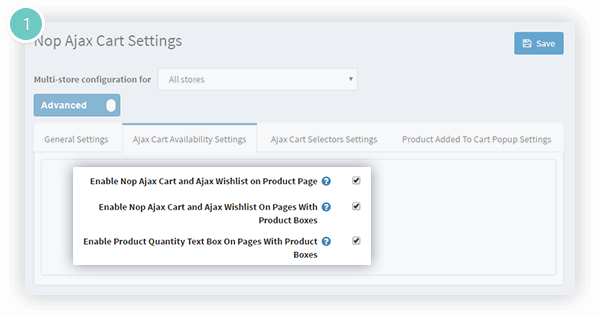This image appears to be a detailed screenshot from an e-commerce platform's configuration settings, specifically within a module related to an AJAX-based shopping cart. At the top left corner of the screenshot, there is a light bluish-green circular icon with a white numeral "1" inside it, outlined in white. 

In the background, there's a header that reads "NOP NOP AJAX CART SETTINGS," indicating the section being configured. Below the header, the text reads "MULTISTORE CONFIGURATION" followed by the numeral "4." A drop-down menu is visible, currently showing the selection "ALL STORES."

On the far right side of the screenshot, a prominent blue tab featuring a floppy disk icon and labeled "SAVE" can be seen, suggesting a save option for settings. Under the "MULTISTORE CONFIGURATION" heading, there's another blue tab on the far left labeled "ADVANCED."

Below this section, four tabs are listed, with the second tab, "AJAX CART AVAILABILITY SETTINGS," currently selected. The other tabs are titled "GENERAL SETTINGS," "AJAX CART SELECTOR SETTINGS," and "PRODUCT ADDED TO CART POPUP SETTINGS."

In the forefront, a white box includes several toggleable options related to the AJAX cart functionality:
1. "ENABLE NOP AJAX CART AND AJAX WISHLIST ON PRODUCT PAGE" - which includes a question mark icon for additional information and is presumably enabled.
2. "ENABLE NOP AJAX CART AND AJAX WISHLIST ON PAGES WITH PRODUCT BOXES" - also enabled.
3. "ENABLE PRODUCT QUANTITY TEXT BOX ON PAGES WITH PRODUCT BOXES" - similarly, this option is enabled.

Each of these settings features a check mark indicating they are currently activated.